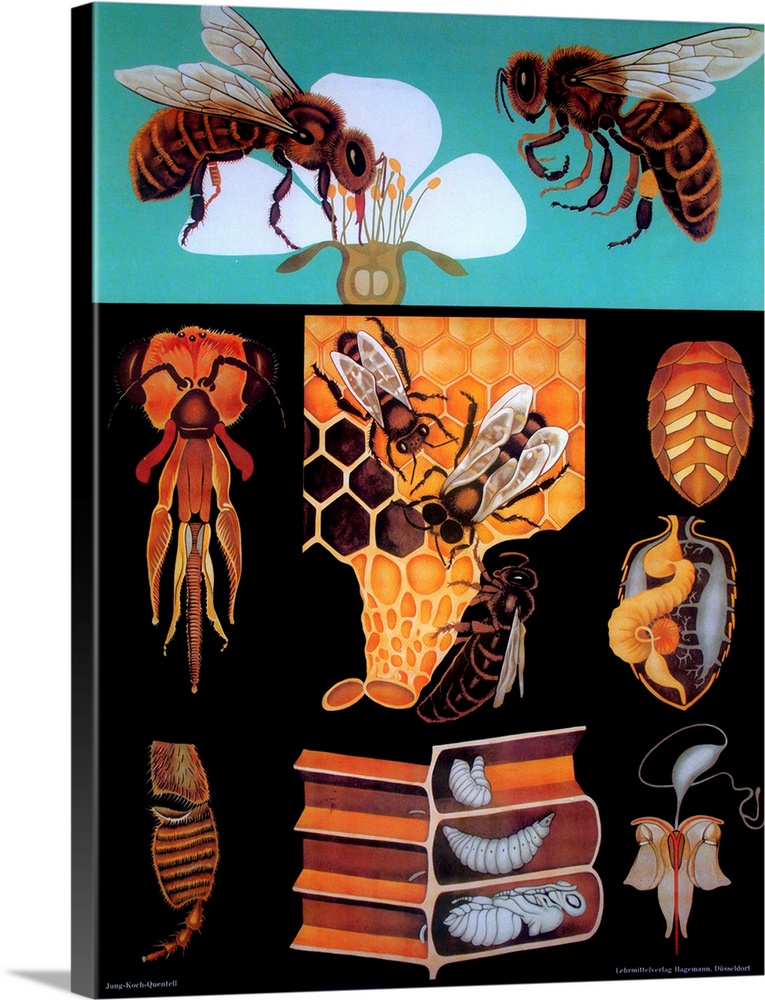This hand-drawn image, possibly a book cover, intricately depicts various aspects of honeybee life and anatomy against a vibrant background. At the top, two honeybees with yellowish-brown furry bodies and large black eyes are shown extracting pollen from a white-petaled flower with a green stalk and yellow pollen, set against a turquoise background. A black section below this showcases detailed diagrams: the head of a honeybee with visible antennae and mouthparts, a half abdomen, and the stinger, along with the inner anatomy including the digestive tract. Further down, three worker bees are actively engaging with a honeycomb, depicted with meticulous attention to their body parts. The bottom section illustrates the developmental stages of a bee larva within the honeycomb, transitioning from larva to mature bee. This educational artwork, rich in color and detail, highlights the different phases and functions of honeybee life, potentially serving as a cover for a scientific book on bees. Small white text appears at the bottom, although it is unreadable in the image.